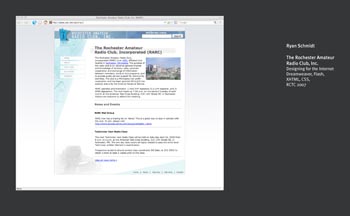The image displays a black rectangle-oriented landscape with a screenshot of a website on the left side and some text on the right. The website screenshot is very small and becomes overly blurry when enlarged, making the text illegible. The upper left corner of the website is shaded light blue, complemented by a medium blue banner stretching across the top. In the upper left corner, a short menu with small white banners overlays the light blue triangle. The website's main text is printed in black, with the header in bold. Certain portions of the text appear in blue, indicating underlined links. Additionally, there is a small rectangular photo of what looks like a building against a blue sky located just to the right of the first paragraph of text.